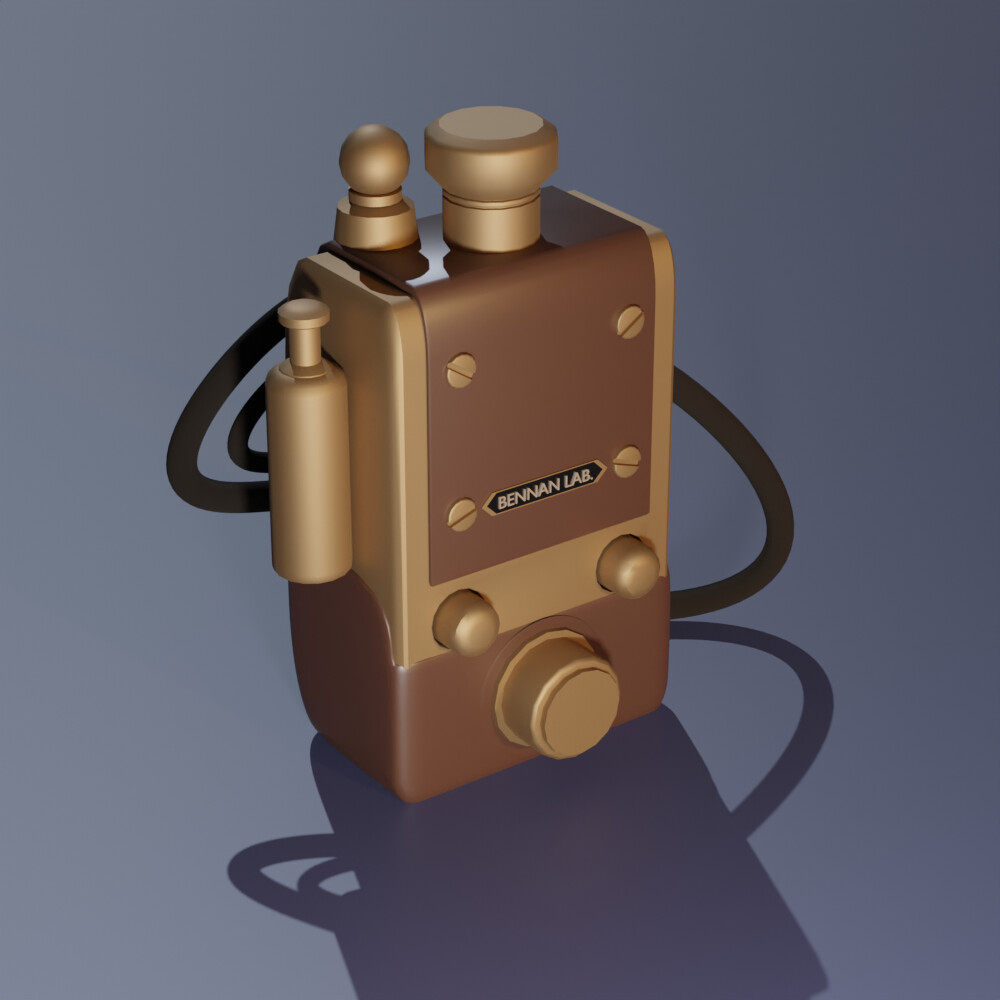The image displays a detailed 3D render of a square, bronze-colored metallic device situated against a bluish-gray to purplish background. The edges of this instrument are rounded, and it features multiple knobs and pressable buttons. Notably, the bottom portion of the device has a brown metal casing, which includes a turnable gold knob. Above this section, within the gold body, are two additional pressable gold buttons. 

At the top, there’s another brown metallic plate fastened by four flathead gold screws, and attached to this plate is a black tab labeled "Brennan Lab" in white text. The left-hand side of the device showcases a cylindrical element with another gold button and some black cables extending from the side and back.

The topmost part of this apparatus displays a snow globe-shaped structure with a golden ball at its base and another gold knob at the top. A leather strap is attached to the back of the machine with four screws, suggesting that it can be hung from the neck or shoulder. The intricate details of the instrument, including the shadows cast in the image, hint at its purpose as a sophisticated gauge or measuring tool.